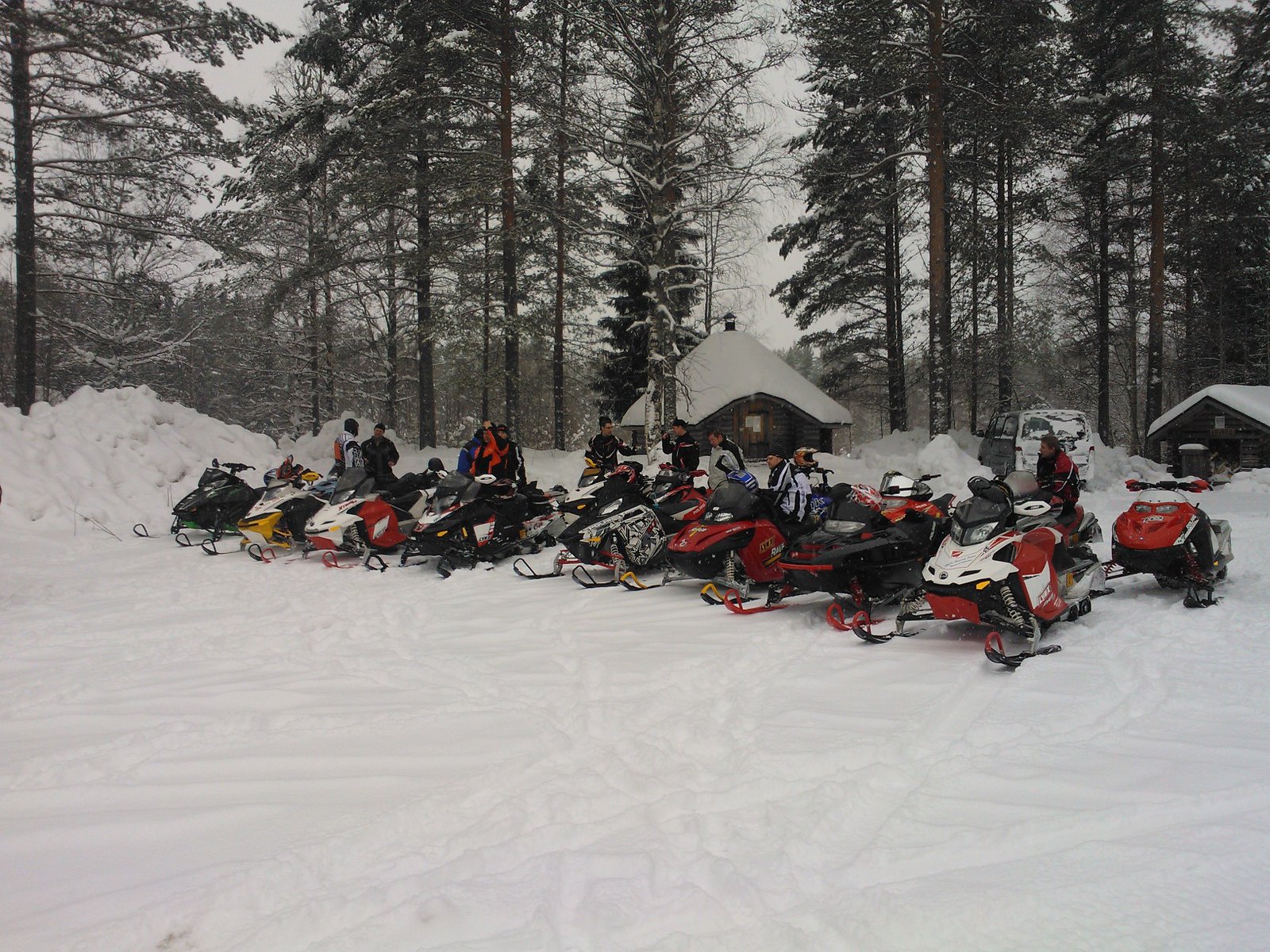This outdoor winter scene captures a group of people preparing for a snowmobile ride against a foreboding gray sky. The ground is blanketed with snow, with large plowed piles to the left and visible snowmobile tracks etched across a flat area. In the background, there are two log cabins, each adorned with thick layers of snow on their A-frame roofs; one cabin has a black metal chimney and a lighted window. A group of fir and pine trees, dusted in snow, rise behind the buildings. The snowmobiles, numbering around ten, are lined up diagonally across the image. They come in various colors and models, including combinations of red, black, white, and yellow. Each snowmobile has people seated on them, dressed in winter gear. The scene suggests either an early morning or dusk setting, enhancing the tranquil yet anticipatory mood of this snowy adventure.